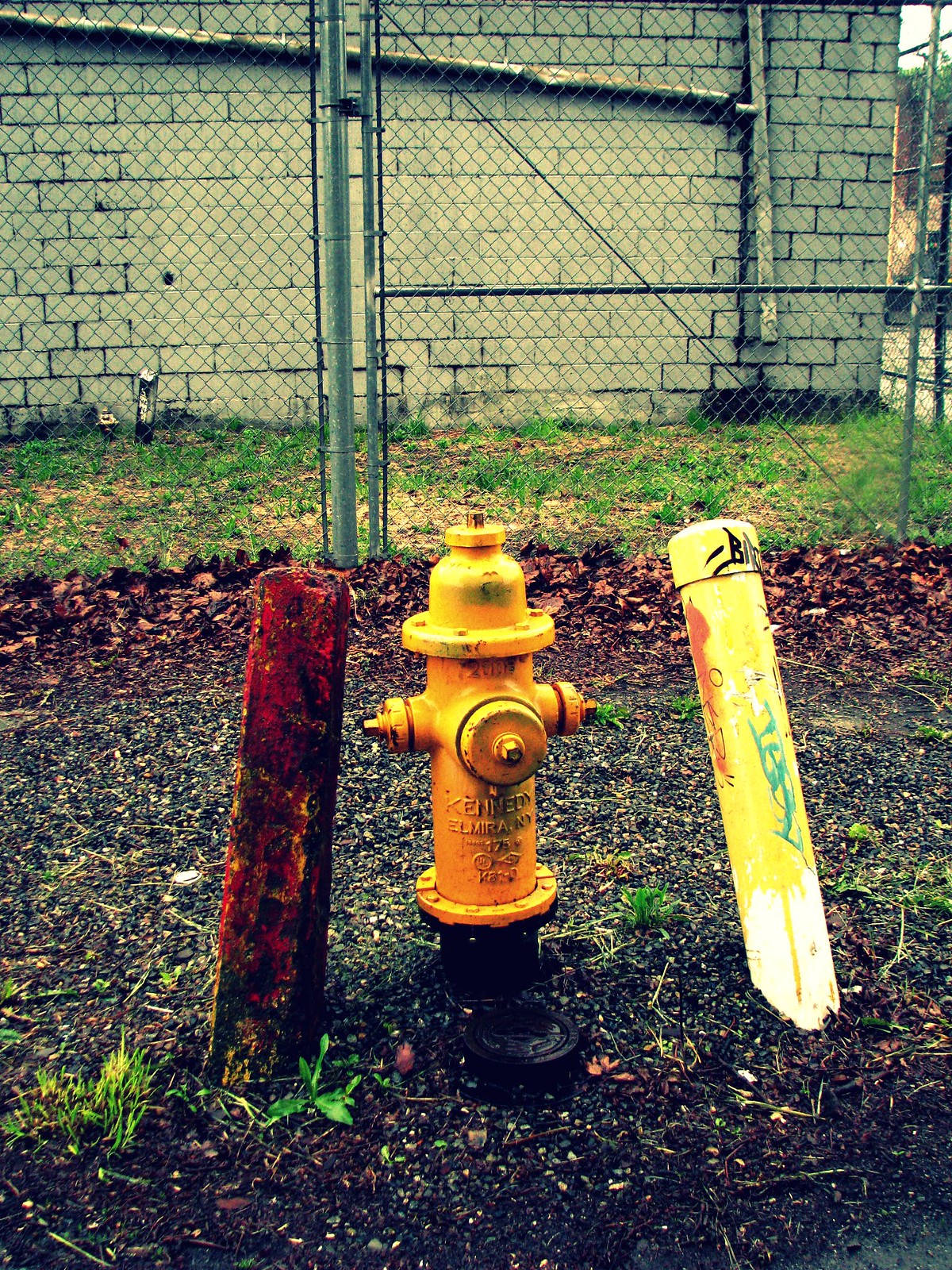This image captures an aged yellow fire hydrant positioned centrally in an outdoor setting. The hydrant's paint is weathered, with noticeable black spots adorning its front and sides, and parts where the top paint has rubbed off. To the left of the fire hydrant stands a shorter concrete pillar, while to its right is a tall yellow post, seemingly made of plastic or PVC, which has been graffitied and capped with a screw top. All three objects are anchored in dirt, interspersed with sparse strands of green grass and scattered dead leaves.

In the background, a tall chain-link fence runs parallel to the trio, its base lined with patches of dark, possibly wet, soil and more dead leaves. Beyond the fence lies a dilapidated white brick building suggesting an overall rundown environment. Complementing the scene are rusty poles leaning to the right and forward, contributing to the aged and neglected atmosphere. The mixture of green and dead grass, muddy rocks, and dry patches further enhances the sense of abandonment and decay in this New York-like setting.